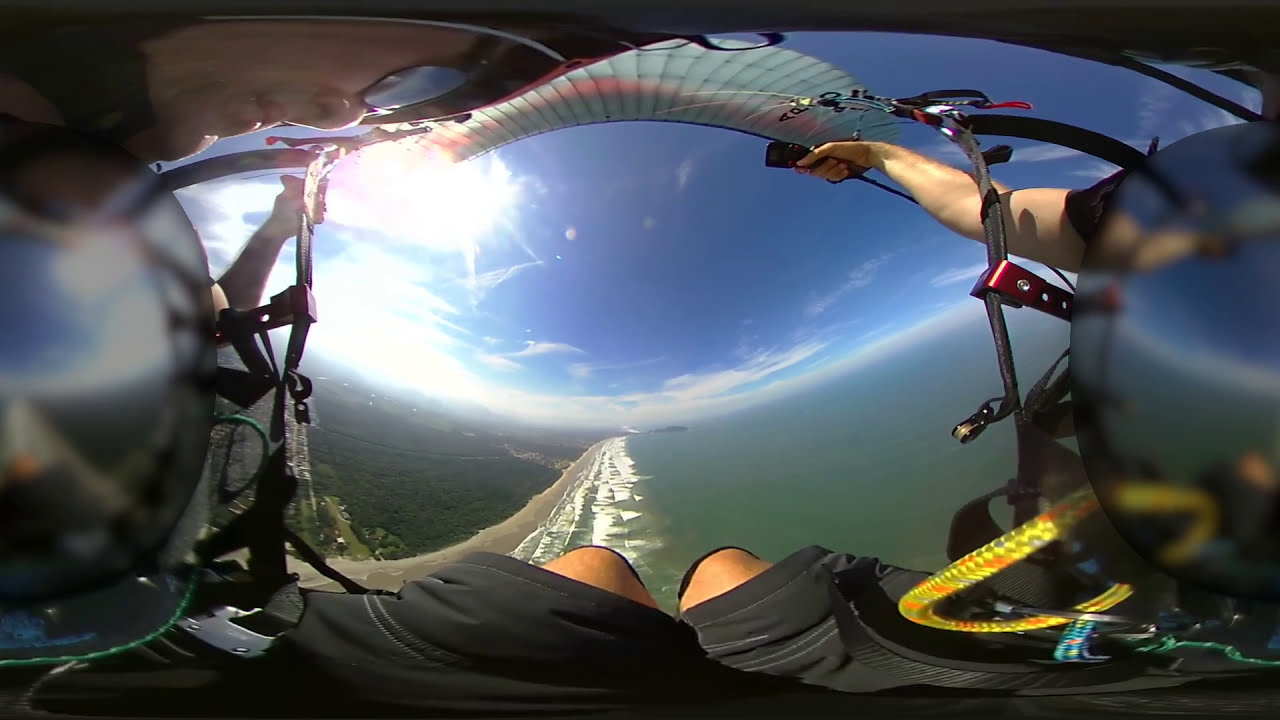The image is a high-resolution digital photograph taken from a first-person perspective, showing a man engaging in parasailing. The man is centrally positioned in the image, with his arms at the top, holding onto the parasailing gear, and his legs visible at the bottom, clad in shorts that reveal his knees. The scene is set outdoors, presumably in the middle of the day, under a blue sky adorned with a few white clouds.

The man appears to be floating approximately 300 feet in the air, high above a picturesque coastline. Below, the beach stretches out with its tan sand kissed by the surf of the ocean waves. To the left, the coastline is bordered by lush green trees, providing a sharp contrast to the deep blue ocean on the right. The photograph showcases a variety of colors including black, brown, yellow, orange, red, gray, blue, tan, green, and white, contributing to the vivid and dynamic nature of the scene. The man is suspended by a parabolic sail that is fully inflated, hinting at either wind propulsion or a small, unseen engine providing thrust. Overall, the image captures the thrilling activity of parasailing against the serene backdrop of nature.